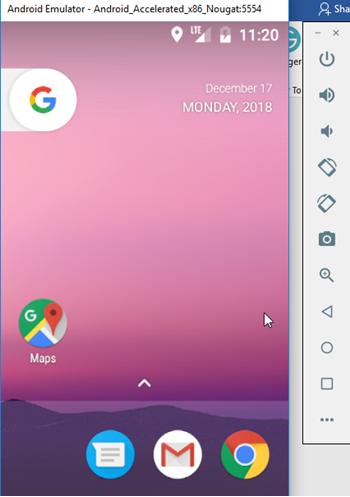A detailed pop-up overlaying a webpage displaying an Android Emulator screen. The emulator showcases an Android Accelerated x86 running Nougat, identified by the virtual device Android_5554. The screen's background features a gradient sky of pink fading into purple, descending into a horizon of deep purple dunes and light purple water. Marked with the date Monday, December 17th, 2018, and the time 11:20, the status bar indicates a half-charged battery with three signal bars. Prominent app icons include the Google and Google Maps logos, accompanied by a bottom row featuring Gmail, Chrome, and Messenger icons. Partially visible behind this pop-up, a sidebar displays various phone-related icons for power, sound, camera, and other functionalities.